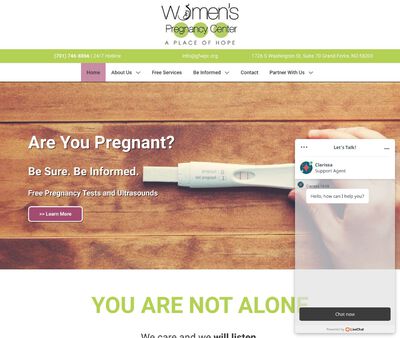The image displays a screenshot of a website predominantly featuring a white and green color scheme. The background consists of a wood-paneled tabletop with a pregnancy test and a young woman's hand on the right side. Superimposed on this background, text reads, "Are you pregnant? Be sure. Be informed. Free pregnancy test and ultrasound," accompanied by a purple button labeled "Learn More."

At the top of the webpage, the header reads "Women's Pregnancy Center: A Place of Hope." The logo includes three green circles behind the words "Pregnancy Center." Below this header, there's a green bar containing contact information, though the font is quite small and difficult to read.

Further down, a white navigation bar lists the following options: Home, About Us, Free Services, Be Informed, Contact, and Partner with Us. The "Home" option is highlighted in a maroon color. At the bottom of the page, green text reads "You are not alone." Additionally, a live chat box is open in the bottom right corner, displaying a message from a support agent saying, "Hello, how can I help you?"